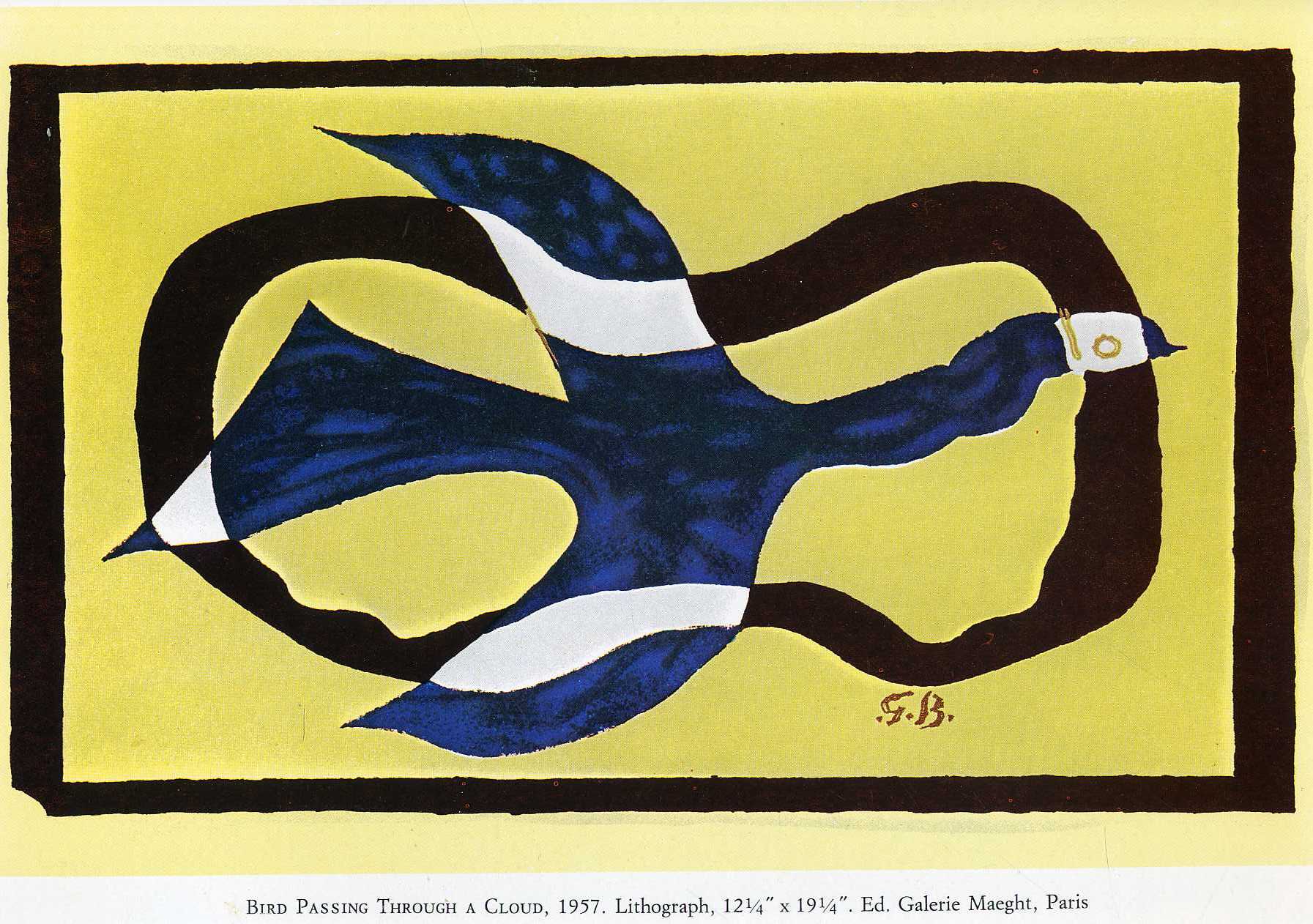The artwork titled "Bird Passing Through a Cloud, 1957" by G.B. is an abstract lithograph framed in brown and set against a white background. Measuring approximately 12.25 inches by 19.25 inches, it is showcased at Ed Gallery Mate in Paris. The piece features a predominantly blue bird with two shades of blue - dark and medium - adorned with white stripes on its wings, a white-tipped tail, and a white face accented by a gold eye. The background is a vibrant yellow, intersected by a peanut-shaped, transparent brown cloud. This abstract composition also includes variations of yellow, particularly lighter shades at the top and bottom borders, and a subtle black oval behind the bird. The entire scene is encased within a dark border, highlighting the bird flying through this fantastical, nature-inspired setting.